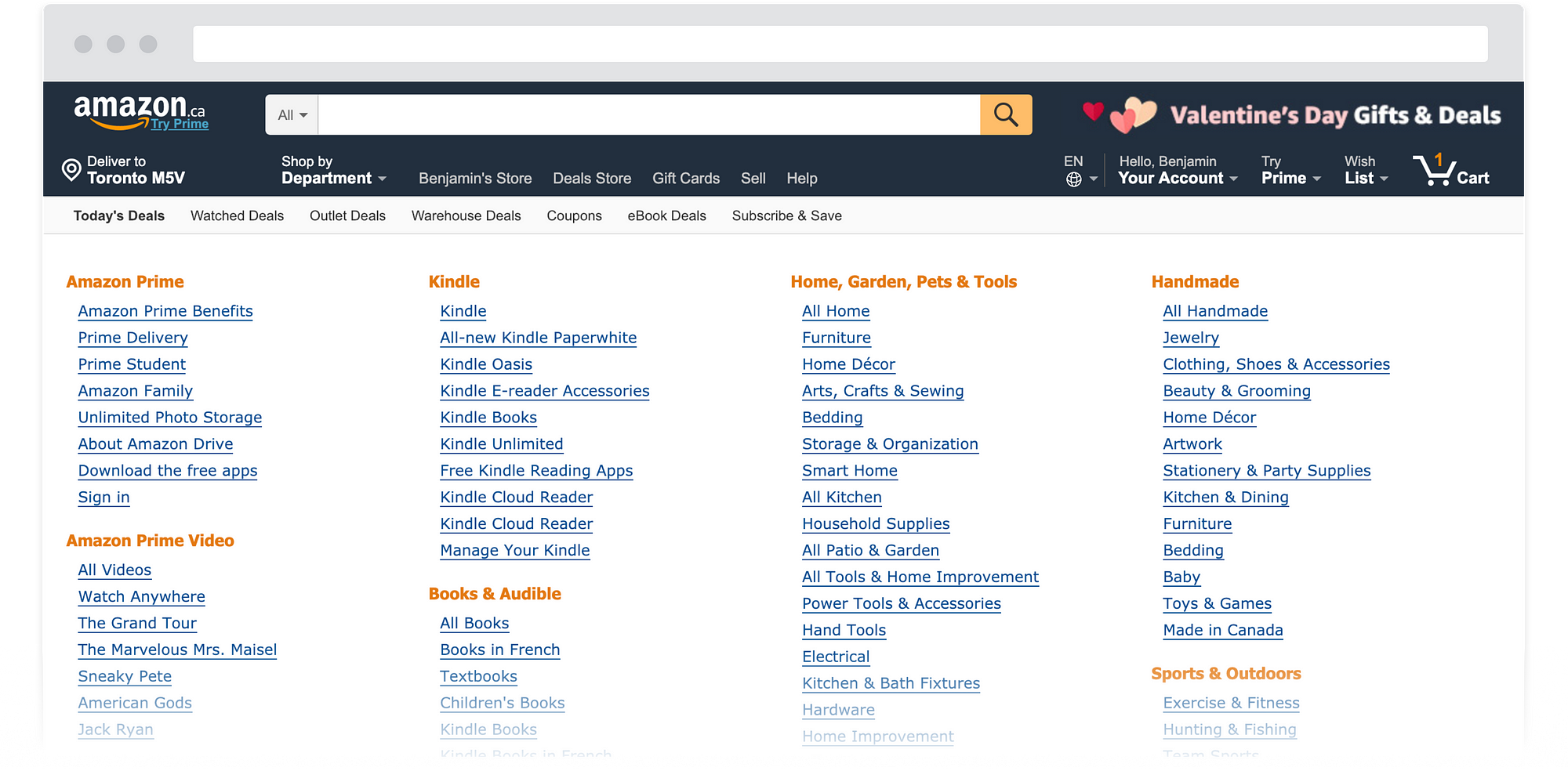The image depicts a screenshot of the Amazon Canada website (Amazon.ca) displayed on a minimalist browser interface. The browser's search bar is empty, highlighting the simplicity of the layout. The page is set to deliver items to Toronto, with the postal code MV5 visible.

At the top right corner of the screen, there is a prominent banner for Valentine's Day gifts and deals, written in a pale pink font for "Valentine's Day" and a white font for "gifts and deals," accompanied by three hearts in red, pink, and beige. On the user section of the page, a greeting reads "Hello, Benjamin," indicating the logged-in user's name. Benjamin has one item in his cart and has not subscribed to Amazon Prime, as evidenced by the "Try Prime" option. The language selected is English.

The page provides links to various Amazon services and categories, including Amazon Prime, Amazon Prime Video, Kindle, Books and Audible, Home Garden, Pets & Tools, Handmade, Sports & Outdoors, and more. However, the full list is partially obscured by a gradient fade at the bottom of the screen.

A white navigation bar at the top features different deal categories, such as "Today's Deals" (the current section), "Watch Deals," "Outlet Deals," "Warehouse Deals," "Coupons," "eBook Deals," and "Subscribe and Save." Additionally, it is suggested that Benjamin may be an Amazon seller given the presence of a store link. The likely timeframe of this screenshot is February, inferred from the Valentine's Day promotional content.